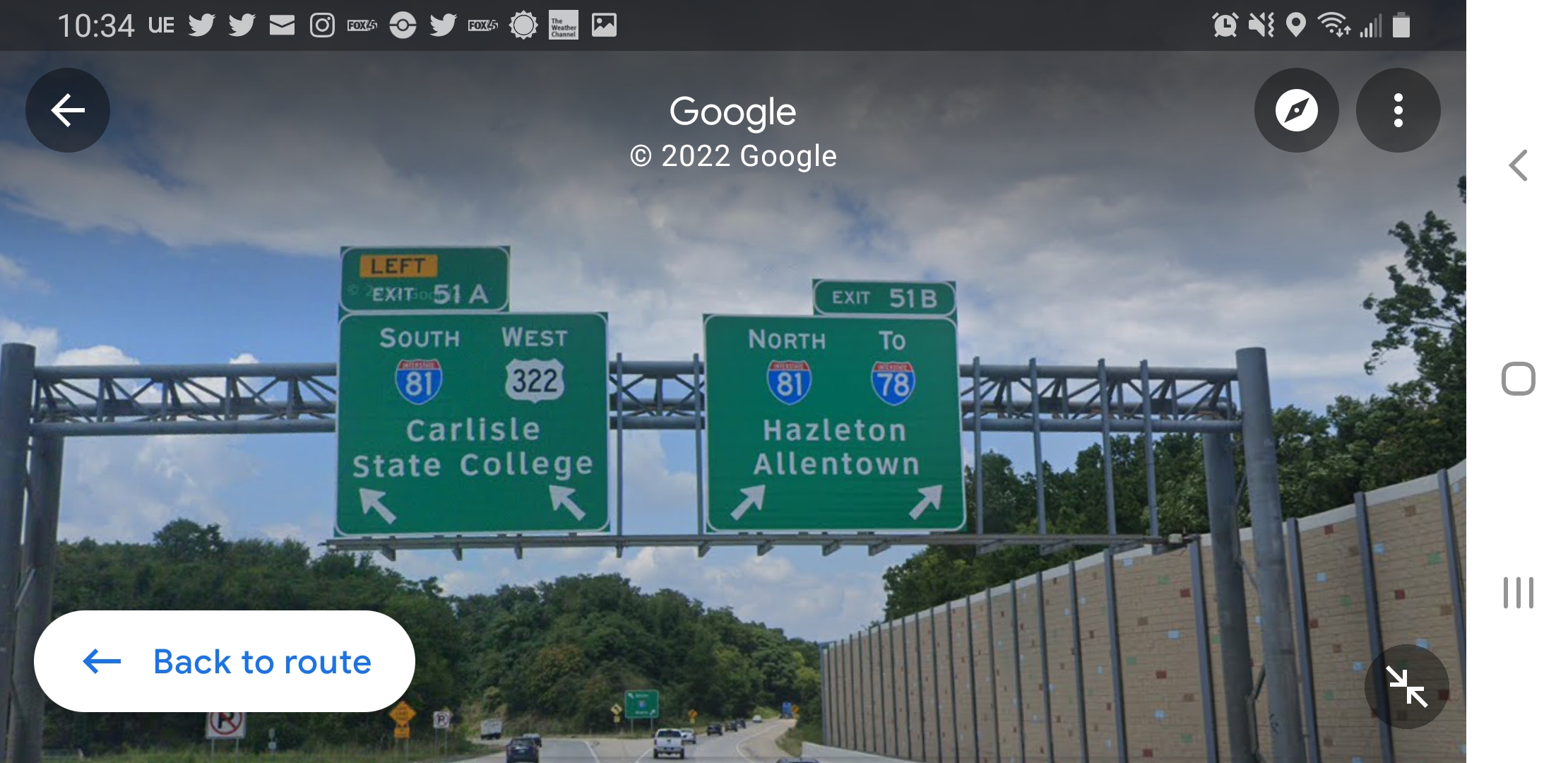This image, likely captured by a Google Street View camera, showcases a bustling intersection captured in a Google Street View calendar. Dominating the scene is a metal scaffolding that supports large, green overhead signs directing interstate traffic. 

On the left, a sign for Exit 51A directs drivers south onto Interstate 81 or west onto Road 322, with clear instructions to head towards Carlisle and State College. This sign features two left-pointing arrows. Adjacent to it, a sign for Exit 51B guides vehicles north onto Interstate 81 towards Interstate 78, with destinations including Hazleton and Allentown, marked by arrows pointing to the right.

In the lower part of the image, the interstate forks into a V shape, enhancing the visual complexity of the scene. The right side of the image reveals a tan sound barrier wall, demarcating the boundary between the interstate and a nearby neighborhood. 

The sky above is mostly cloudy, with patches of blue peeking through, casting a subdued light over the scene. Surrounding the interstate, lush green trees add a touch of natural beauty to the otherwise urban setting.